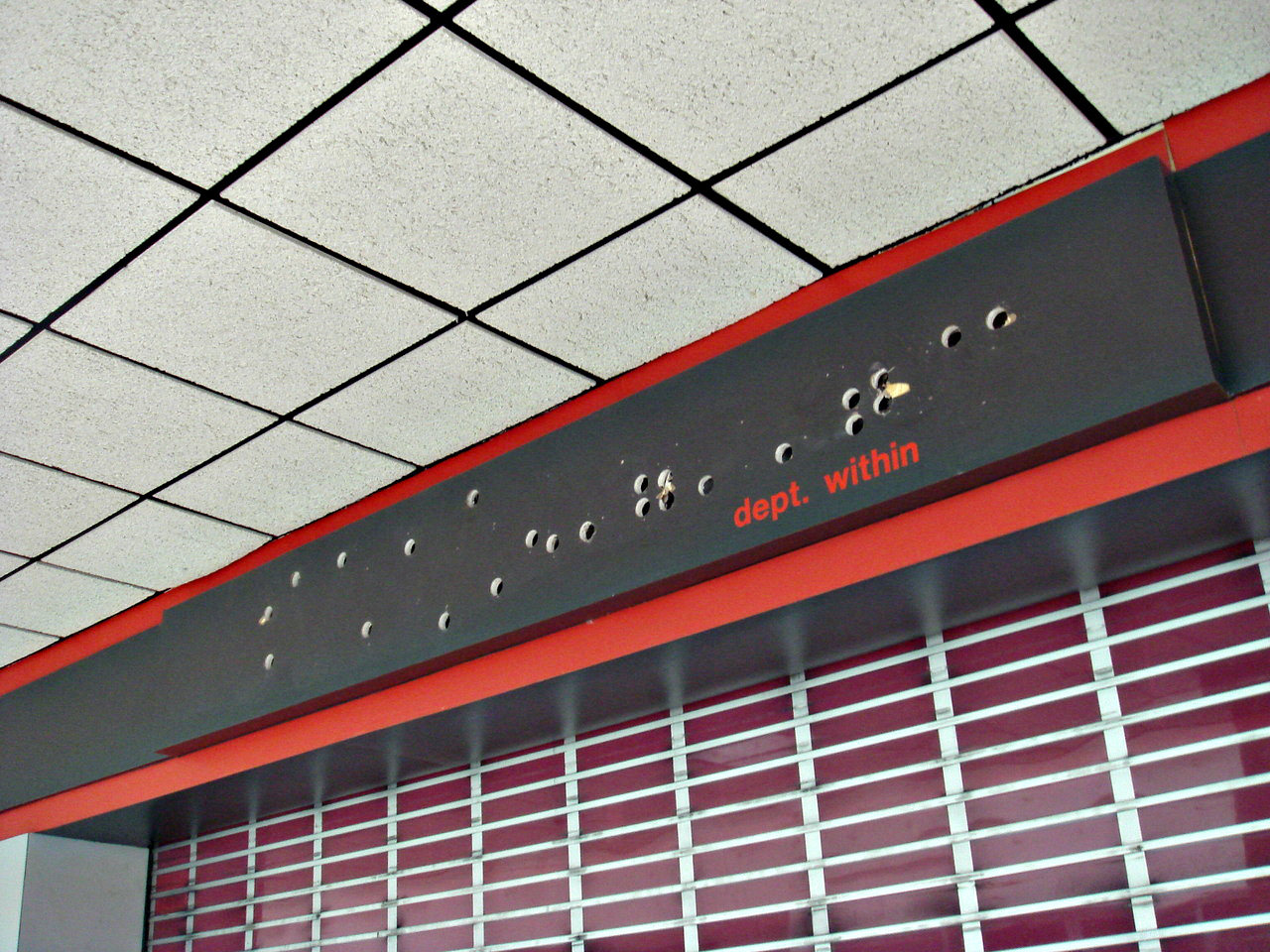This photo depicts the inside of a shopping mall, focusing on a closed-down store. The ceiling features white tiles outlined in black. At the center, a metal gate is pulled down, inactivated, indicating the store is no longer operational. Behind the metal gate is a solid red surface obstructing any view into the interior. To the left side, there's a silver-grey area adjacent to the gate. Above the entrance, a rectangular sign features a black background with red lettering that reads "DEPT.within." The sign bears numerous holes, likely remnants of mounts for previous signage. The scene reflects a space that has been vacated, with the once active shopping area now silent and inactive.